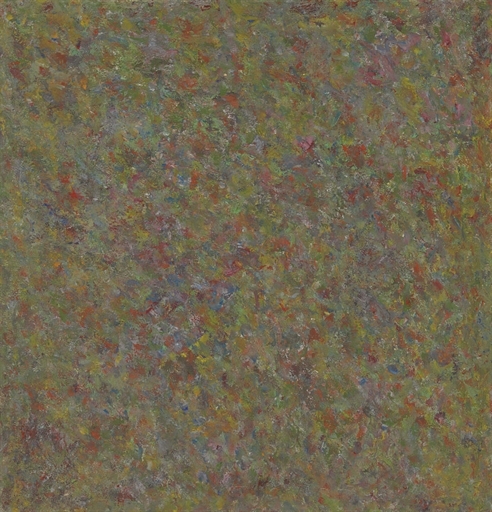This image is an abstract painting characterized by random splashes of various colors with no discernible shapes or patterns. The palette is vibrant and diverse, featuring prominent hues such as purple, blue, green, yellow, red, and brown. Notably, darker colors like gray and blue are heavily concentrated in the center, while lighter shades, including yellow, green, and orange, dominate the edges. The painting evokes a sense of chaos with its seemingly haphazard assortment of colors layered and intermingled, reminiscent of a wild, unstructured collage of paint. Despite the lack of defined forms or imagery, the artwork captivates with its dynamic interplay of colors and textures.